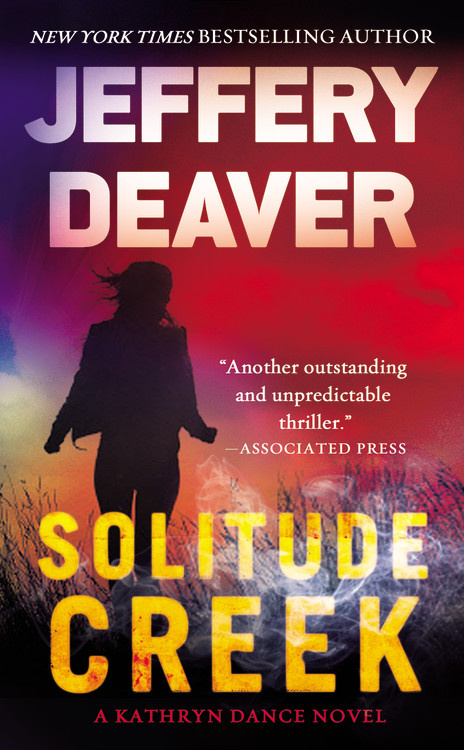The cover of the book is a compelling and atmospheric scene. At the very top, in white lettering, it proudly states "New York Times Bestselling Author." Beneath that, in bold, large white capital letters, the author's name stands out: "Jeffrey Deaver." The background of the cover transitions from a dark field of tall grass at the bottom to a striking sky filled with shades of dark red, fuchsia, orange, yellow, and purple stretching from right to left. In this dramatic backdrop, the silhouette of a woman is prominently featured, appearing as a shaded black outline that suggests detail without revealing specifics. On the right side of the book cover, there is a review in white text that reads, "Another outstanding and unpredictable thriller" by the Associated Press. At the bottom, the title "Solitude Creek" is displayed in large, bold yellow font. Just below that, in red capital letters, it indicates, “a Catherine Dance novel.”